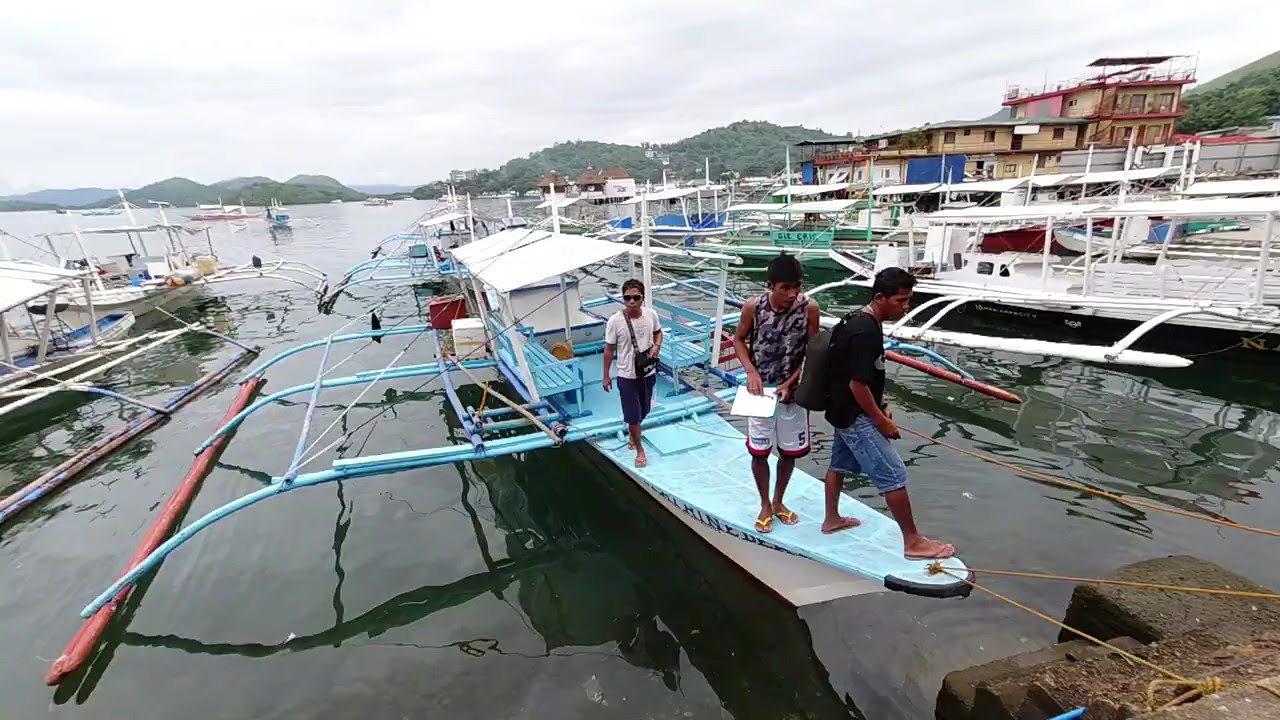In this detailed image, we see a bustling dock made of stone or cement bricks, where 12 long, narrow boats resembling elongated surfboards with small canopies are tethered. Each boat, akin to a slender kayak or catamaran, features skeletal metal structures on the sides that support buoyant logs, contributing to the vessel's stability. Three young men are seen disembarking one of these specialized boats, distinguished by its light blue hue and red pontoons, under a white roof supported by poles. The boat they are on, tied with yellow cords, has bench seating and is moored to the stone dock at the bow. Surrounding the dock, the green and murky water hints at a lively yet perhaps less maintained harbor, complemented by a backdrop of various boat storage facilities and moored boats. Additionally, a tan, three-story building with patches of blue tarp and red trim can be seen in the background, under an overcast sky filtering diffused sunlight.